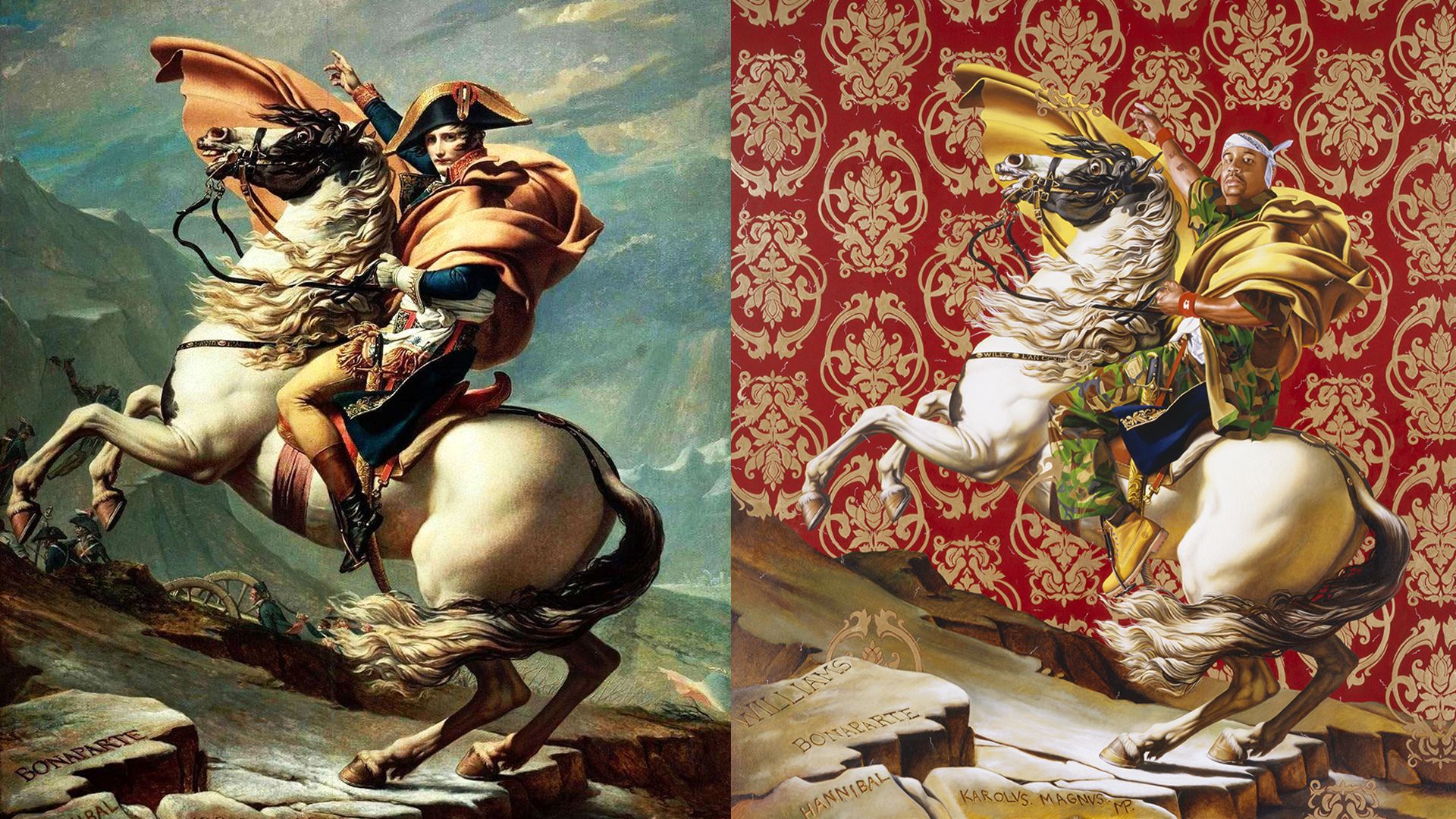The image depicts two men on horseback in near-identical poses. On the left, we have a figure that appears to be Napoleon Bonaparte, dressed in a flowing brown cloak and a tricorn hat, holding his right arm up in direction. He is mounted on a white horse with a yellowish tint, rearing up on a rugged, rocky cliff background with mountains behind him. The rock at the bottom of this image bears the inscription "Bonaparte."

On the right, another image mirrors the pose and scene but with significant variations in details. This figure has darker skin, a beard surrounding his mouth, and wears a white headband and multi-colored garb reminiscent of a dashiki, accompanied by tan hiking boots. His horse is a brighter pure white, also rearing. The backdrop here is a red banner with gold naturalistic designs instead of the mountainous landscape. Notably, rocks in this image feature inscriptions: "Williams, Bonaparte, Hannibal, Carus Magnus." Elements of the red patterned backdrop extend over parts of the rocky base. Both horses’ manes and the men's cloaks appear to be caught in a breeze, enhancing the sense of dynamic movement toward battle.